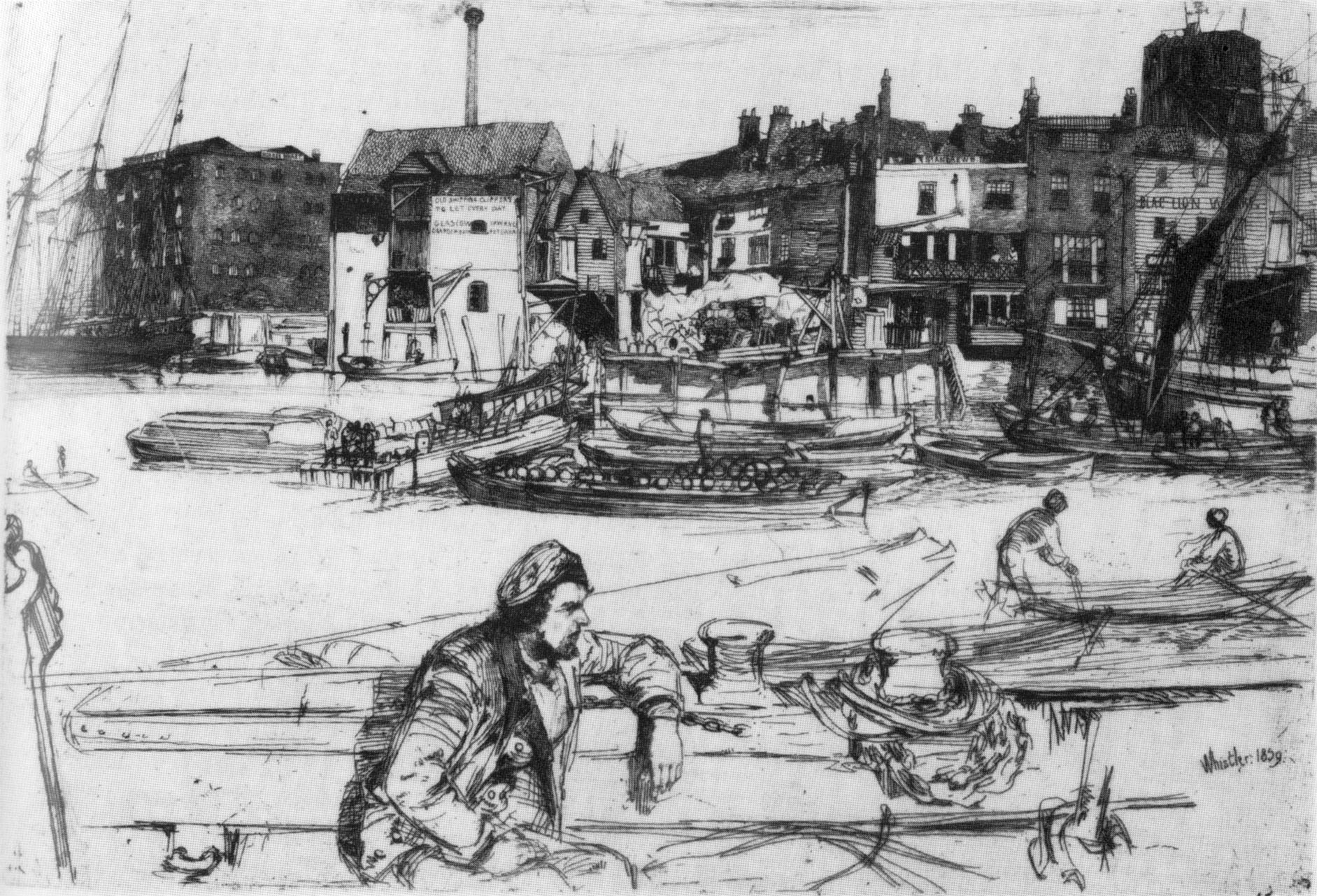The image is a highly detailed, black and white pencil or charcoal drawing set on a letter-size sheet of paper. It depicts a bustling town by the water, with multiple docks and boats. In the immediate foreground, a bearded man wearing a coat and a shipperman's hat sits with his arm resting on a boat by the dock. To his right, two abstractly drawn people are seen rowing a boat. Further into the background, various boats, including 1800s-style paddle and shipping boats, are anchored along the shoreline amongst taller buildings. In the bottom right corner, the drawing is signed with handwritten lettering that reads "Whistler, 1859."